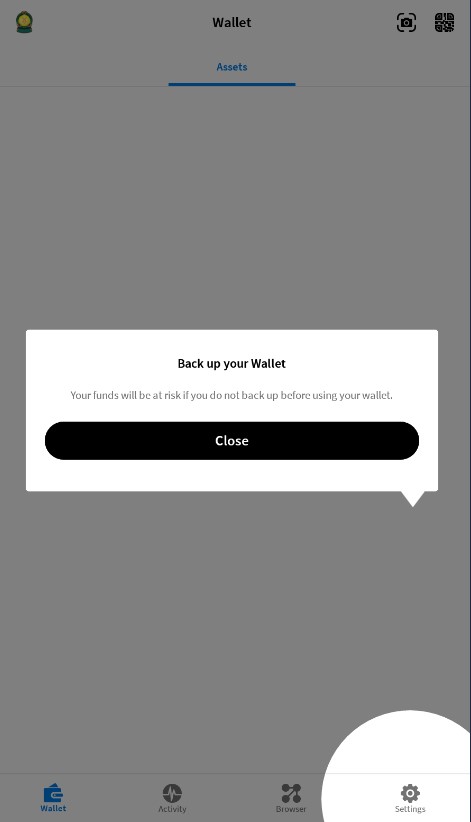This screenshot displays a mobile wallet application in a user interface that emphasizes the importance of backing up wallet data. Dominated by a prominent backup notification in the center, the screen alerts the user with the message: "Back up your wallet. Your funds will be at risk if you do not back up before using your wallet." This alert is enclosed in a clear box with a black 'Close' button featuring white text at the bottom right of the notification.

The top background showcases the word "Wallet" in bold black text, and below it resides a blue button labeled "Assets." Positioned in the upper right corner of the screen is a camera icon, accompanied by several other unrecognizable icons hinting at additional functionalities.

At the very bottom of the screenshot, the navigation bar contains four key icons: a blue "Wallet" icon on the far left, which is clearly selected; an "Activity" icon depicted as a monitor; a "Browser" icon featuring interconnected circles; and a "Settings" icon on the bottom right. The "Settings" button, distinguished by a classic gear symbol, is encased within a large white circle, further highlighted as a key feature of the interface.

Notably, the entire background image is subtly gray to emphasize the overriding backup notification, ensuring that users do not proceed without acknowledging and addressing the warning to safeguard their funds.